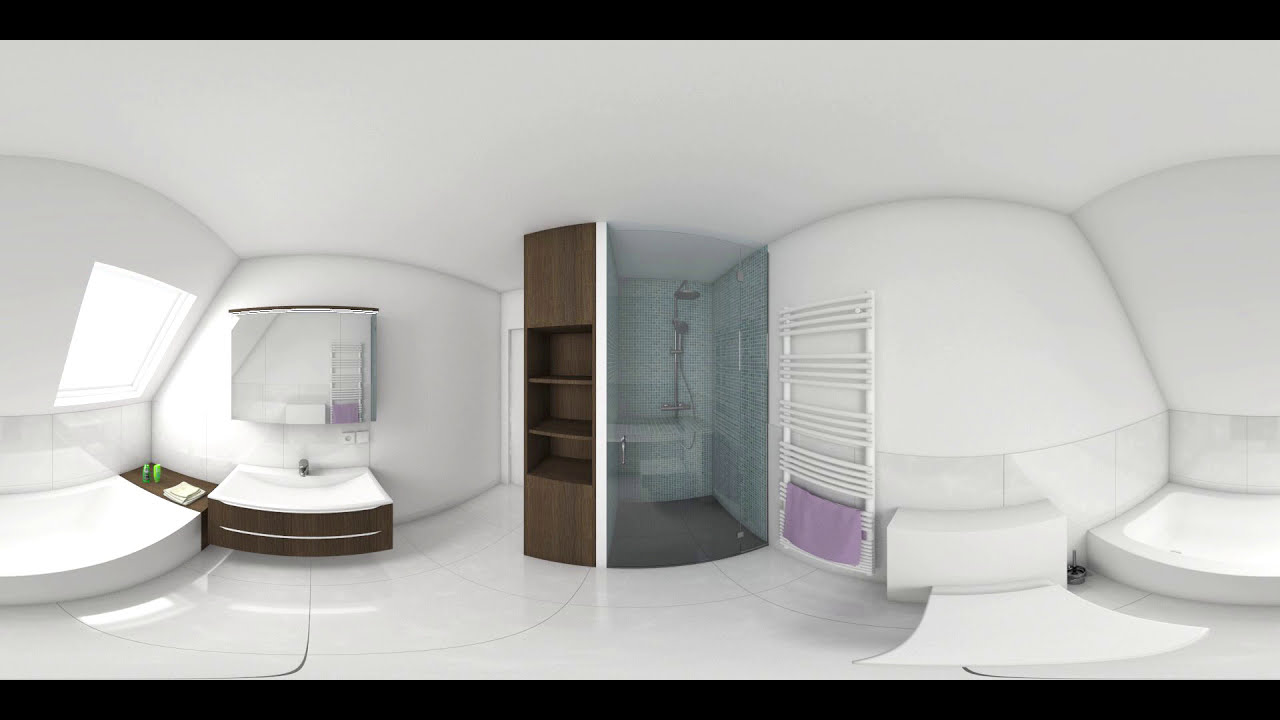The image depicts a modern bathroom with predominantly white walls and surfaces. In the center stands a shower enclosed by a glass door, featuring greenish-blue tiles inside and a dark gray floor. To the left of the shower, a dark brown wooden storage cabinet with three shelves stands next to a wash sink, which has a surprisingly low height but a large basin, with a mirror mounted on the wall behind it. A small window on the left wall allows light to stream into the room. Adjacent to the glass door on the right is a white towel rack currently holding a purple towel at the bottom. Additionally, there is a white bathtub on the right side of the image, slightly recessed into the ground, with a wood front panel. The floor is covered with sleek white tiles, adding to the bathroom's modern aesthetic.